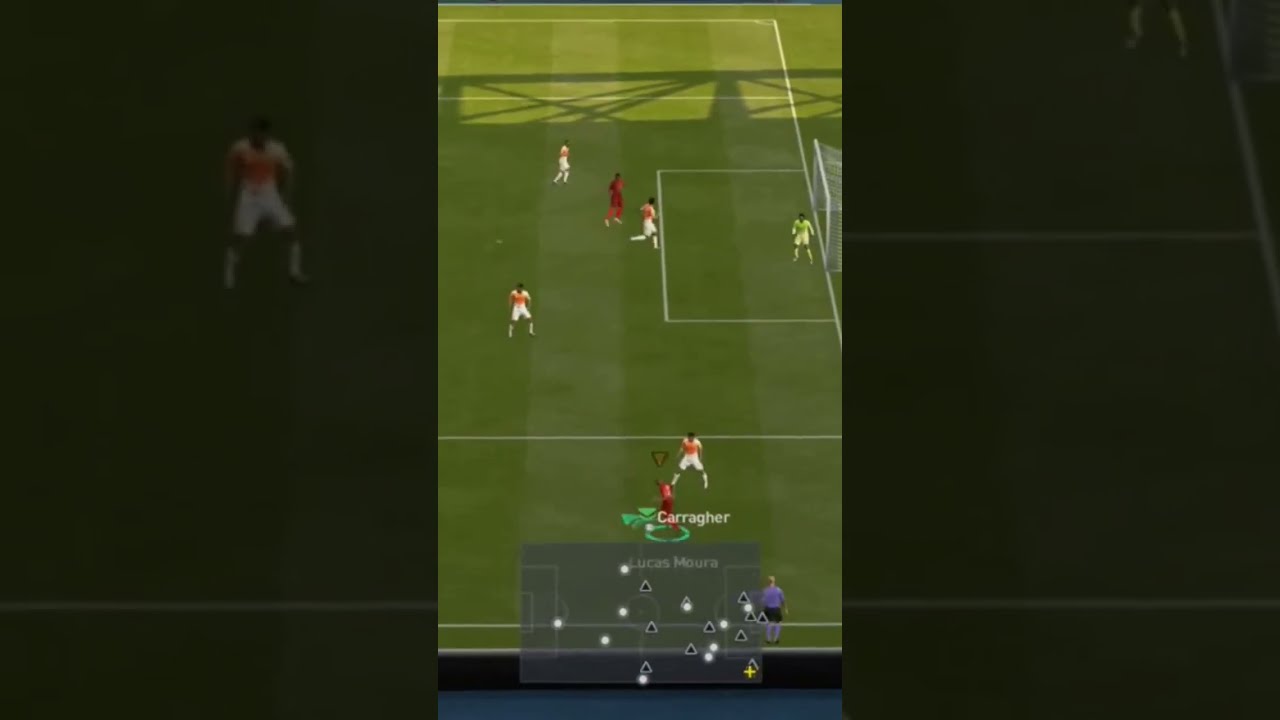The image is a vertical, cell phone-style screenshot from a computer soccer game, captured at an angle of approximately 40 to 50 feet elevation. At the center, the green soccer field is intersected with white lines and dominated by players in distinct uniforms: four in orange and white, two in red, and one in green, identified as Tagoldee. Notably, on the right side of the field, a player in a green uniform stands facing downward near the goal, while another in red, labeled Carragher, is marked by a green circle and an overhead triangle. Nearby, a player in purple is seen on the sideline.

The bottom of the screen features a large, semi-transparent black rectangle displaying a map with white dots and black triangles, likely representing player positions. The field is mostly shadowed, except for the sunlit top edge. The image is additionally framed by zoomed-in segments of the field on both sides, which have a dark black tint that makes them hard to discern. The background of the image is a blurred and faded zoomed-in portion of the main scene, enhancing the overall depth and focus of the gameplay.